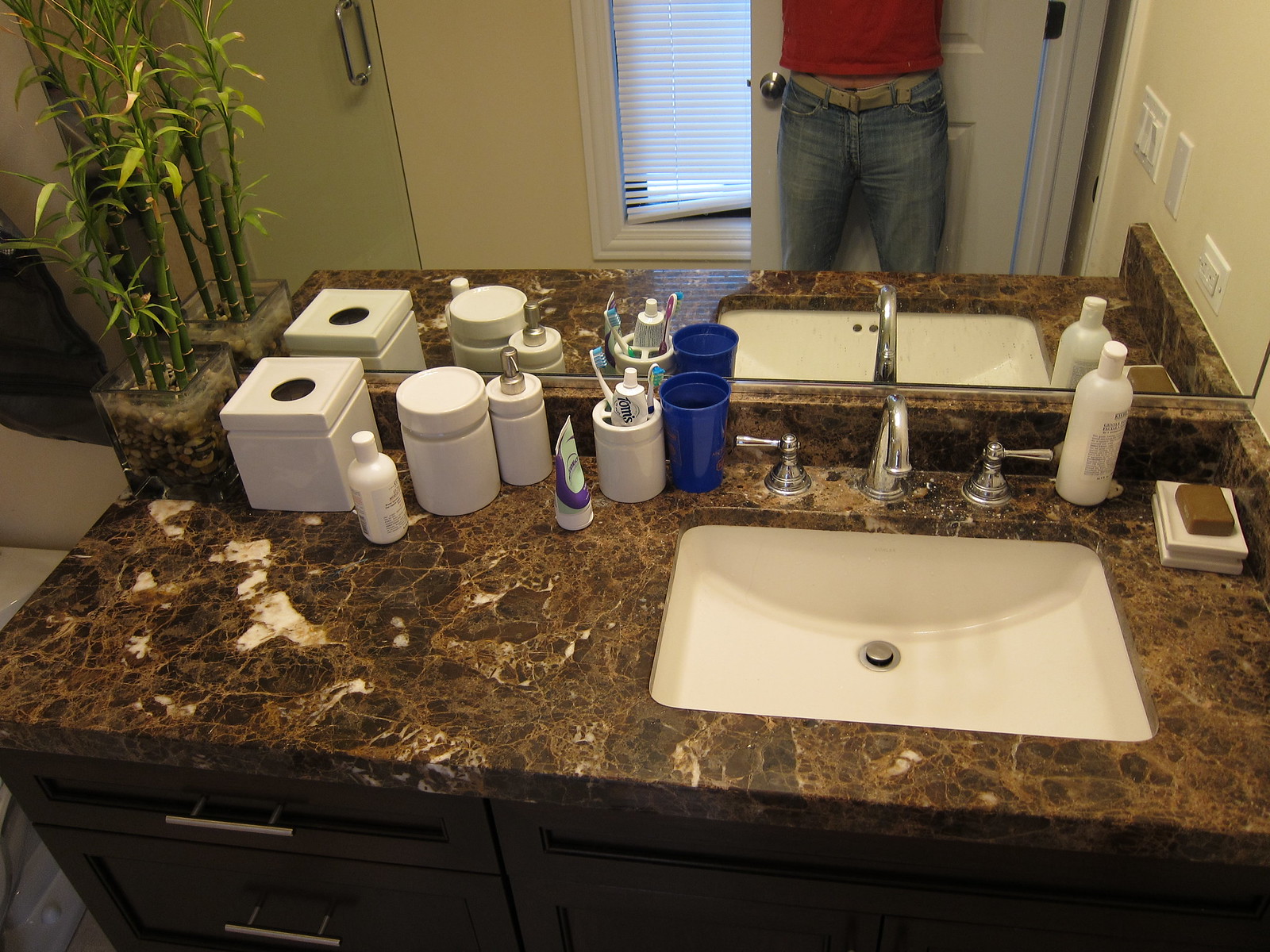The bathroom counter features a predominantly brown granite countertop, adorned with light brown lines and subtle white specks. To the right, a rectangular sink with a slightly open drain is fitted with a sleek silver faucet and matching handles, each with a knob pointing in opposite directions. Adjacent to the sink on the right side is a white squeeze bottle with a white cap, alongside a white soap dish holding a brown bar of soap. 

On the left side of the counter, there is a blue cup. Next to it, a white cup contains a toothbrush and toothpaste. A colorful squeeze bottle with purple and green accents is also present, along with a collection of containers with white caps. A white bottle with a twist-off cap and a white box with a black hole on top are seen nearby. An adjacent black flower pot, transparent in design, displays green-leafed plants shooting upwards.

In the background, a mirror reflects a person wearing blue jeans, a light tan belt, and a red shirt. They stand in front of a door. To their left, a window is partially covered with white blinds that are broken at the bottom.